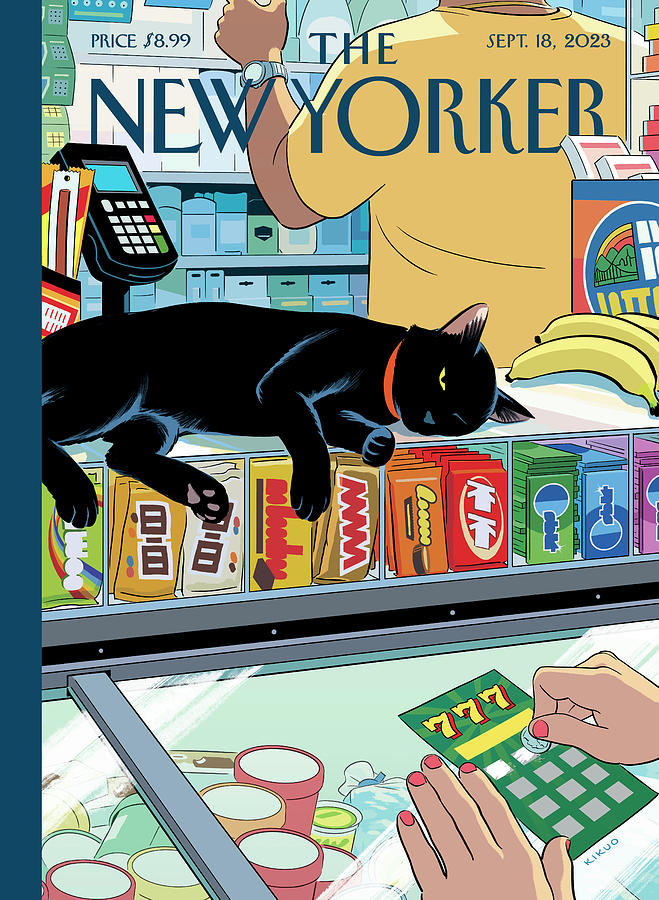The cover of the New Yorker Magazine, dated September 18, 2023, features a detailed illustration of the inside of a convenience store. The store is bustling with various items and activities. At the register, a black cat is lounging atop a display stocked with popular candies such as Skittles, M&M's, Whoppers, Twix, Reese's, Kit Kats, and Orbit Gum. Next to the cat lies a small bunch of bananas. Below the candy display, there is an ice cream cooler with a transparent top, where a woman is intently scratching off a 777 lottery ticket. In the background, a store attendant, dressed in a yellow shirt, is turned away from the register, presumably arranging items on the shelves, with cigarettes visible behind him. Additional details include a credit card machine, a box of beef jerky, and the price of the magazine, marked at $8.99, in the top left corner.